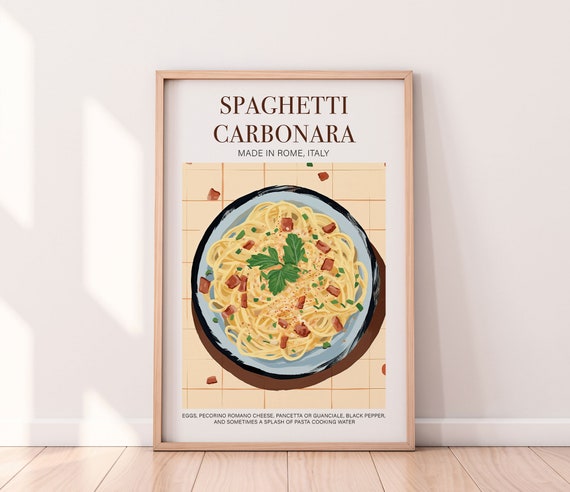This photograph features a rectangular, light brown wooden photo frame placed on a light wood-planked floor against a white wall. The frame contains a white poster with dark brown text at the top, reading "Spaghetti Carbonara made in Rome, Italy." Below the text is a detailed illustration of a circular, white plate filled with cream-colored spaghetti. The spaghetti is topped with green parsley leaves and surrounded by small, brown food pieces, likely pancetta or guanciale, indicative of the traditional Carbonara dish. Behind the plate, a tan-colored background resembling a tablecloth adds a subtle grid pattern to the depiction, complementing the overall white and beige color theme of the setting.